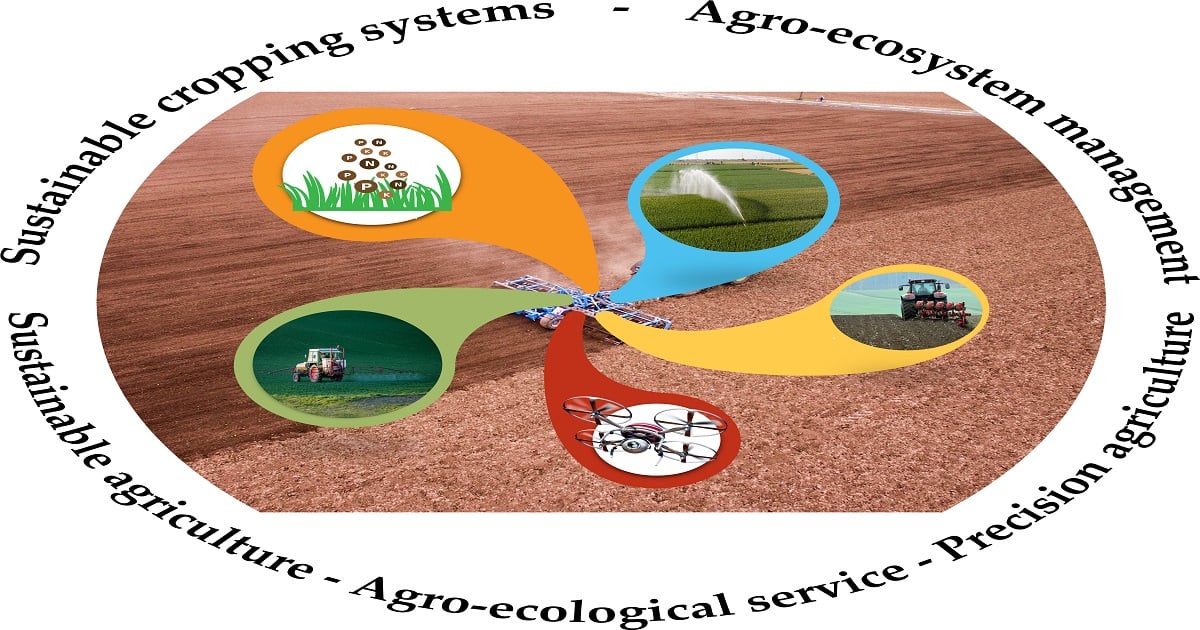This detailed business logo features a central image of a combine tractor harvesting crops in a large field. Surrounding this central combine are various smaller images, forming a swirl pattern that merges into the tractor scene. These smaller images include: another tractor navigating a lush, green pasture; a drone hovering with its four rotors clearly visible; an irrigation system spraying water over crops; and a secondary piece of farm equipment crossing freshly tilled soil. These images are designed to represent different aspects of agriculture and technology. 

The circular shape of the logo extends to the edge, where a ring of text is written in black on a white background, encapsulating core concepts such as "Agro-Ecosystem Management," "Precision Agriculture," "Sustainable Agriculture," "Sustainable Cropping Systems," and "Agro-Ecological Service." The edge of the logo unifies these themes, indicating the company’s holistic and innovative approach to modern farming practices.

Each section within the circle is color-coded with "petals" that resemble a flower: an orange petal with grass and embedded letters, a blue petal with a sprinkler, a yellow petal with farm equipment, a red petal with a drone, and a green petal with a tractor. These elements blend agricultural imagery with technology and sustainability concepts, capturing the essence of the company’s commitment to precision and sustainable farming solutions.